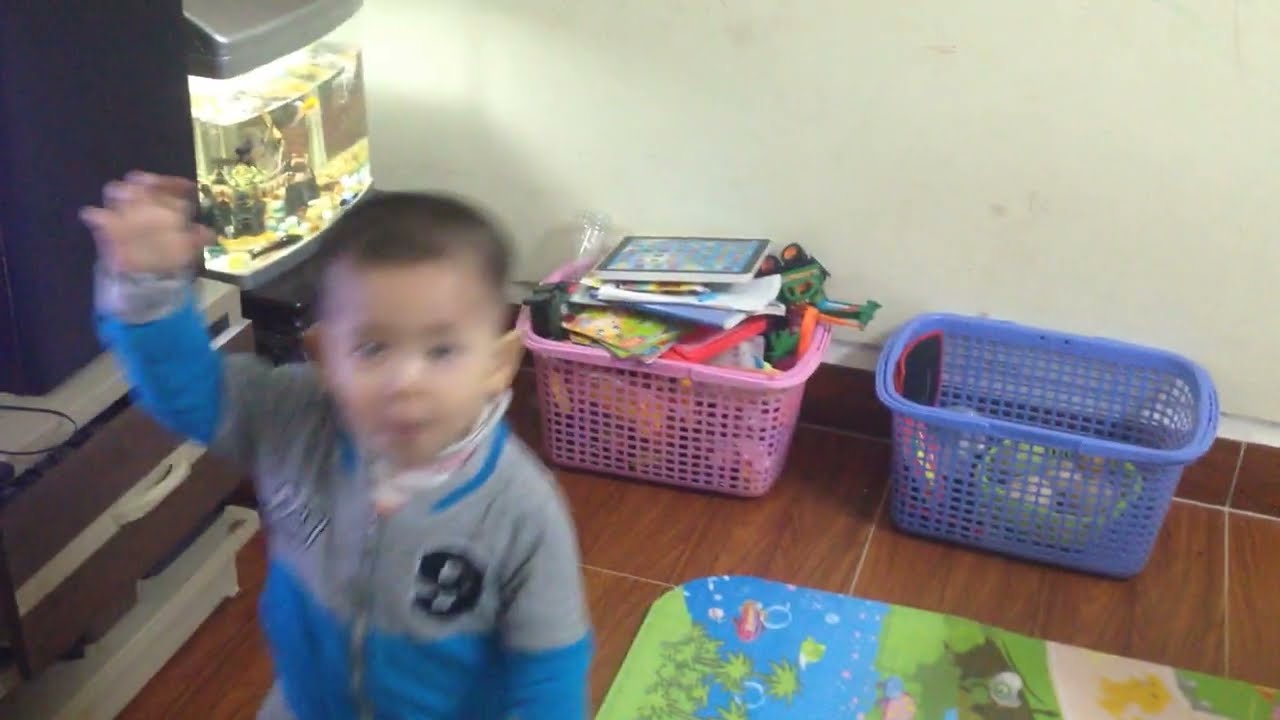The image captures a playful scene in a child's room. A young, likely Asian toddler with short black hair is situated on the left side of the frame. He is blurry, indicating movement, as he looks towards the camera with his right arm raised. He wears a gray and teal zip-up jacket, adorned with the number nine. The backdrop features wooden floors and white walls. To the left, there's a small aquarium with fish, providing a cozy maritime touch. On the wooden floor behind him, two rectangular baskets are visible. The pink one is overflowing with toys and books, while the blue one is a third full with additional toys. Near the bottom right corner of the image, a colorful play mat is partially visible, adding to the room's lively atmosphere.